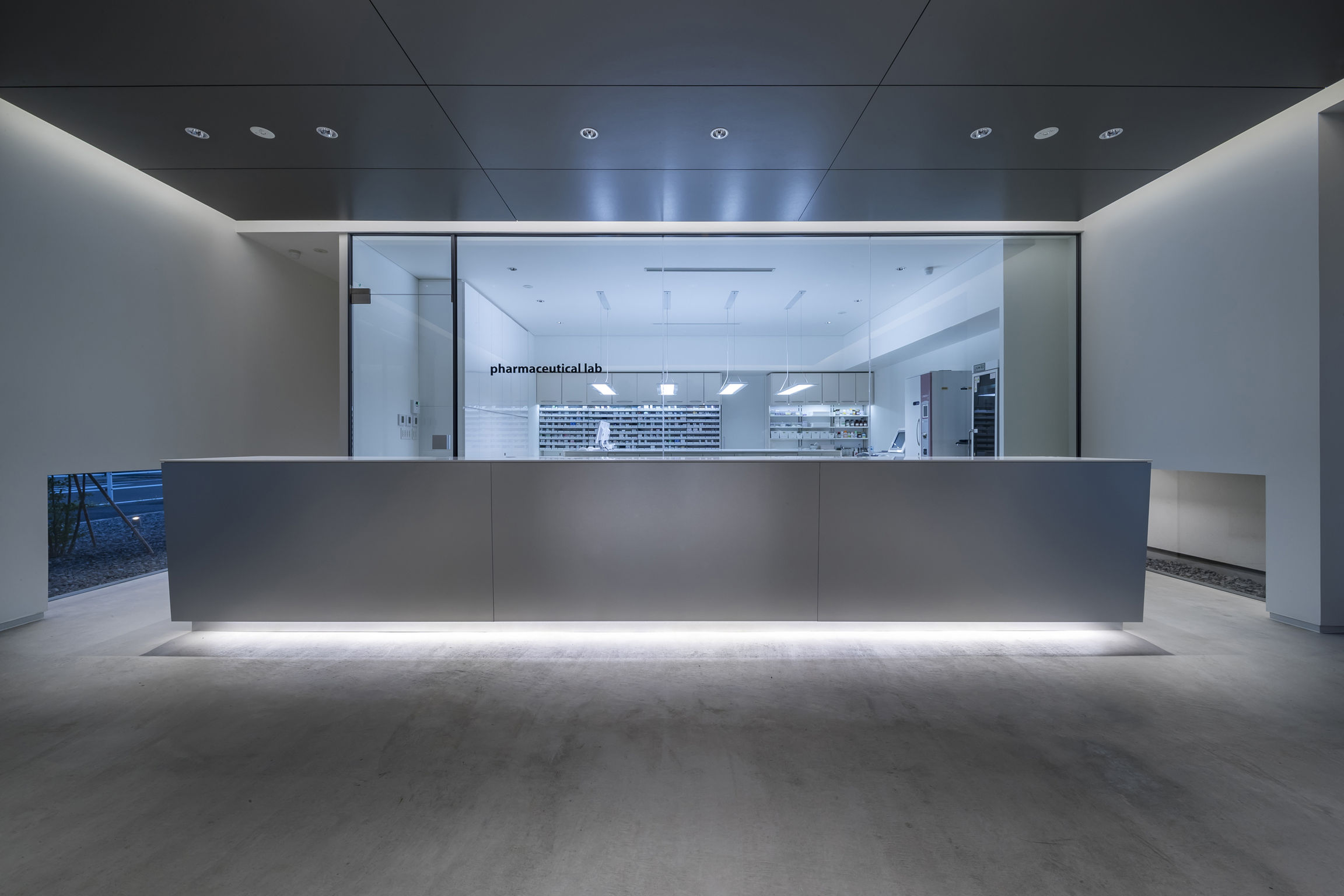The image portrays a modern, empty laboratory viewed from a likely hallway or waiting area. Dominating the foreground is a long, silver-colored horizontal barrier illuminated with white light from beneath, set against a gray and light gray floor. Beyond this barrier is a large glass window bearing the black text "Pharmaceutical Lab" on its left side. Flanking this central window are columns of glass, with the right column tinted light gray and the left column tinted light blue. The ceiling, composed of nine black panels delineated by black lines and featuring small holes for lighting, boasts three lights each on the left and right sides, and two in the middle. Blue light reflects off this ceiling, enhancing the modern ambiance. Visibly, the back wall of the lab has cabinets and standing shelves, although much of the interior detail is obscured by the central barrier.